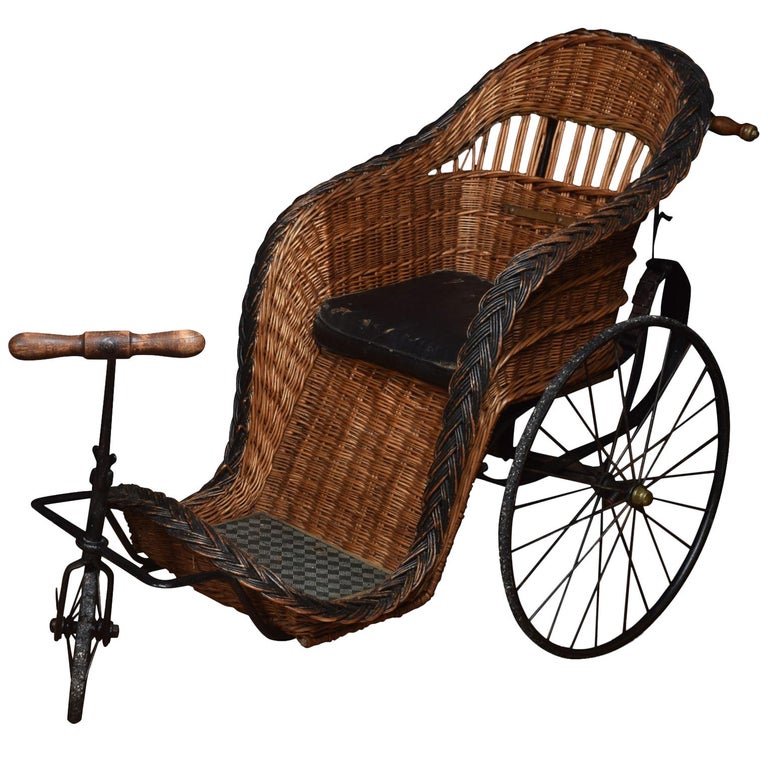This image depicts an antique vehicle, likely from the late 1800s or early 1900s, which appears to be an old-fashioned wheelchair or a type of wicker carriage. The vehicle is crafted with a combination of black metal and brown wicker, evoking the appearance of a wicker chair mounted on a tricycle frame. Dominated by these two colors, the black elements consist of the metal parts, including the seat frame and wheels, while the brown segments include the wicker seating and potential painted wicker details that exhibit a dark brown hue.

The contraption features three wheels: a smaller wheel in the front, equipped with a steering handle, and two larger wheels on either side, reminiscent of a horse and carriage design. However, the image shows only the right side wheel in detail. This device includes a floor segment for resting feet, integrated with the wicker seating area that provides a vintage, grandmotherly aesthetic.

The precise function of this vehicle is ambiguous. While there are handles at the back suggesting that it might be pushed by another person, there is no clear evidence of pedals, implying it might not be self-propelled like traditional bicycles. The front steering handle, connected to the small wheel, implies a potential for manual steering, albeit not easily accessible if seated normally. Overall, the item seems to straddle the line between a tricycle and a manually pushed wheelchair, with its distinctive, woven wicker design making it a unique historical piece. The image has no background, giving the impression that the object was copied and pasted from a textbook or similar source.